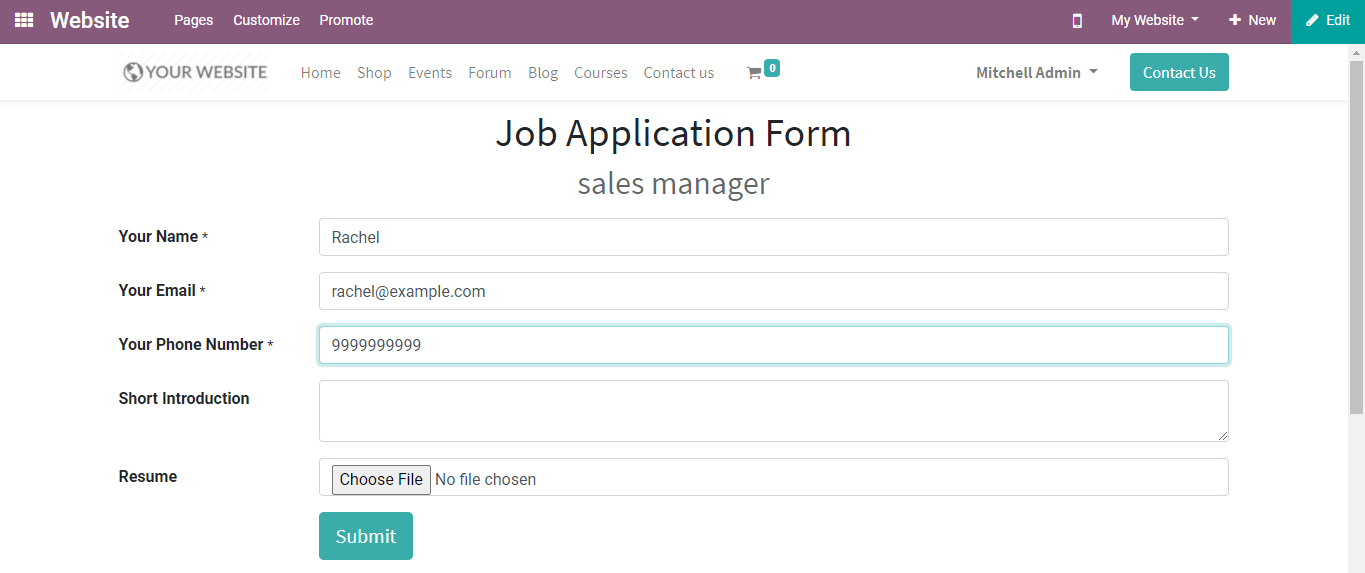This screenshot depicts a website builder interface with a predominantly violet top bar stretching horizontally across the page. The bar features an insignia composed of nine small squares arranged in a grid, adjacent to the word "Website" written in white. Main navigation headings such as "Pages", "Customize", and "Promote" are prominently displayed in the white font.

On the right-hand side of the bar, a picture of a smartphone is shown next to the label "My Website," accompanied by a dropdown arrow, a plus sign for creating new elements, and a green pencil icon labelled "Edit" in white letters against the green background.

Below the bar, additional navigation options are listed under the header "Your Website" next to a globe icon. These options include "Home", "Shop", "Events", "Forum", "Blog", "Courses", "Contact Us", and a green shopping cart icon indicating zero items currently in the cart. To the right of these options, the name "Mitchell Admin" appears with a dropdown arrow, and a green "Contact Us" button is displayed in white letters below it.

Centrally positioned on the page, large text reads "Job Application Form" with "Sales Manager" directly beneath it. The form includes various fields: "Your Name," pre-filled with "Rachel"; "Your Email," pre-filled with "Rachel@example.com"; "Your Phone Number," filled with a placeholder of ten nines; a "Short Introduction" text box left blank; and an attachment option labeled "Choose File," indicating no file has been chosen. The form ends with a green "Submit" button.

This detailed visual and textual representation provides a comprehensive overview of the website builder's interface and a specific job application form in progress.